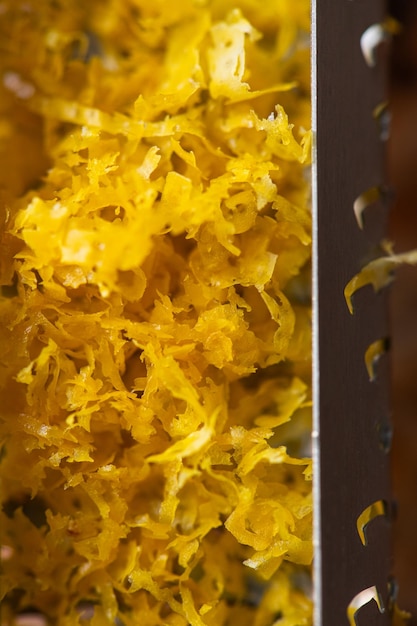This highly detailed close-up image is divided into two vertical sections, showcasing the meticulous process of grating lemon zest using a metal grater. On the left side, the bright yellow lemon zest is seen in fine, thin ribbons, still adhering to the grater and creating a visually striking pattern. The zest appears almost feather-like or leaf-like in texture, adding a delicate contrast to the metallic surface. The right side focuses on the vertically standing grater itself, revealing its silvery-brown, metal body. A distinct detail is the small amount of lemon zest caught in one of the grater's holes, providing a sense of realism to the image. The entire photograph is sharply angled, giving a dynamic perspective and emphasizing the textured interplay between the lemon zest and the grater. The image is set against a clean white background, enhancing the vivid colors and fine details of the grater and zest, though it remains ambiguous whether the setting is real or digitally created.